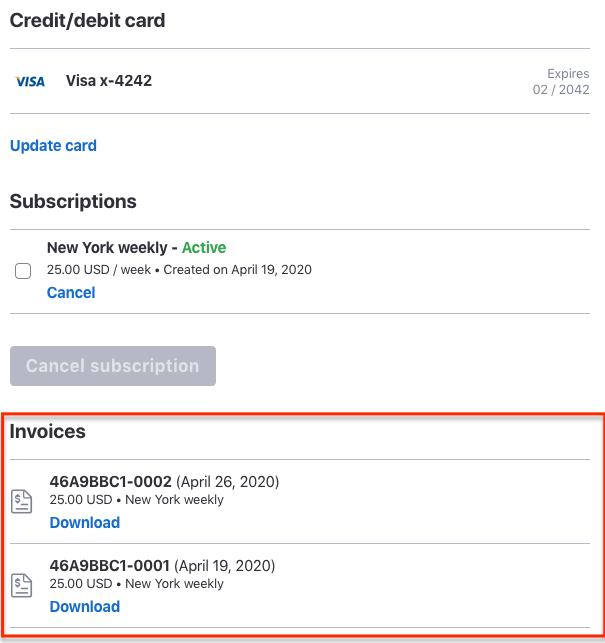In this detailed screenshot, we are viewing the account subscription page for the New York Daily. The primary focus is on the billing information associated with a Visa credit card, with all but the last four digits (4242) obscured for security. The subscription, which remains active, costs $25 USD per week and was initially set up on April 19th, 2020.

The interface provides several actionable options: users can continue the subscription at the current rate, cancel it using a prominent blue button, or update their payment method to a different card if desired. Further down the screen, there are downloadable invoices available for review. These include an invoice dated April 26th, 2020, from the New York Weekly, also billed at $25 USD, and another from April 19th, 2020, for the New York Daily.

In summary, this detailed subscription management page allows the user to:
- Continue or cancel the $25 USD per week subscription.
- Update the payment method currently listed.
- View and download past invoices, such as those from April 19th and April 26th, 2020.
- Cancel the subscription entirely through an additional checkbox option to the right of the screen.

This screen offers a comprehensive overview and considerable flexibility in managing the New York Daily subscription.